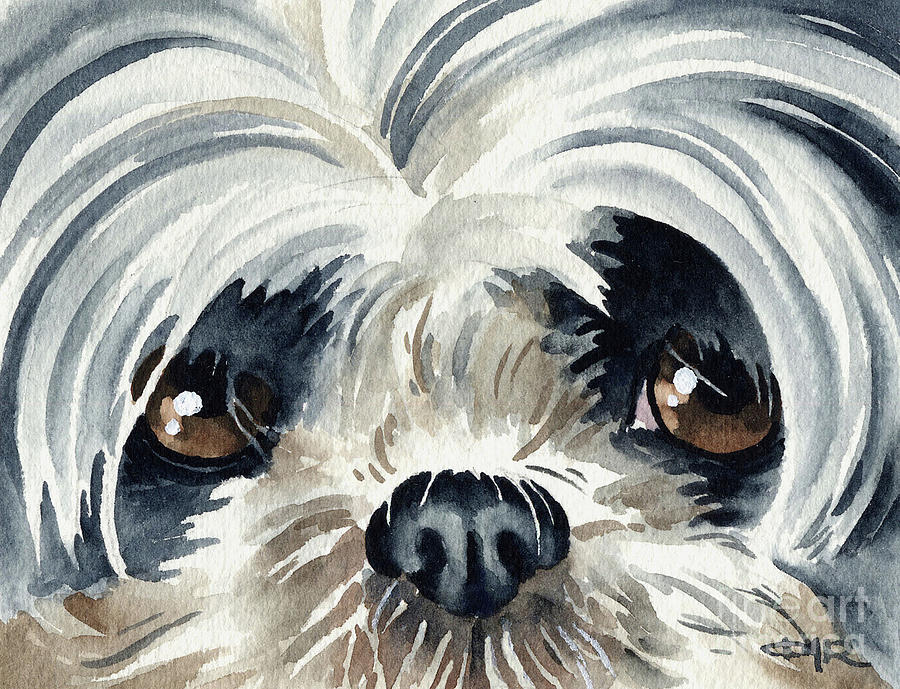This is an up-close watercolor painting of a Shih Tzu dog by artist David Rogers. The painting concentrates on the dog's expressive face, showcasing its large, soulful brown eyes and small black nose. The fur around the dog’s snout is white, while the areas extending outward from its eyes are shaded in a dark charcoal gray. The fur gives the impression of bushy eyebrows and tends to frame the eyes heavily. Additionally, a faint watermark in white or gray reads "The Art America" in the bottom right corner, alongside the artist's signature "D.R." The painting captures a neutral expression with a hint of sadness in the dog's eyes, emphasizing the intricate details of its fur and facial features.